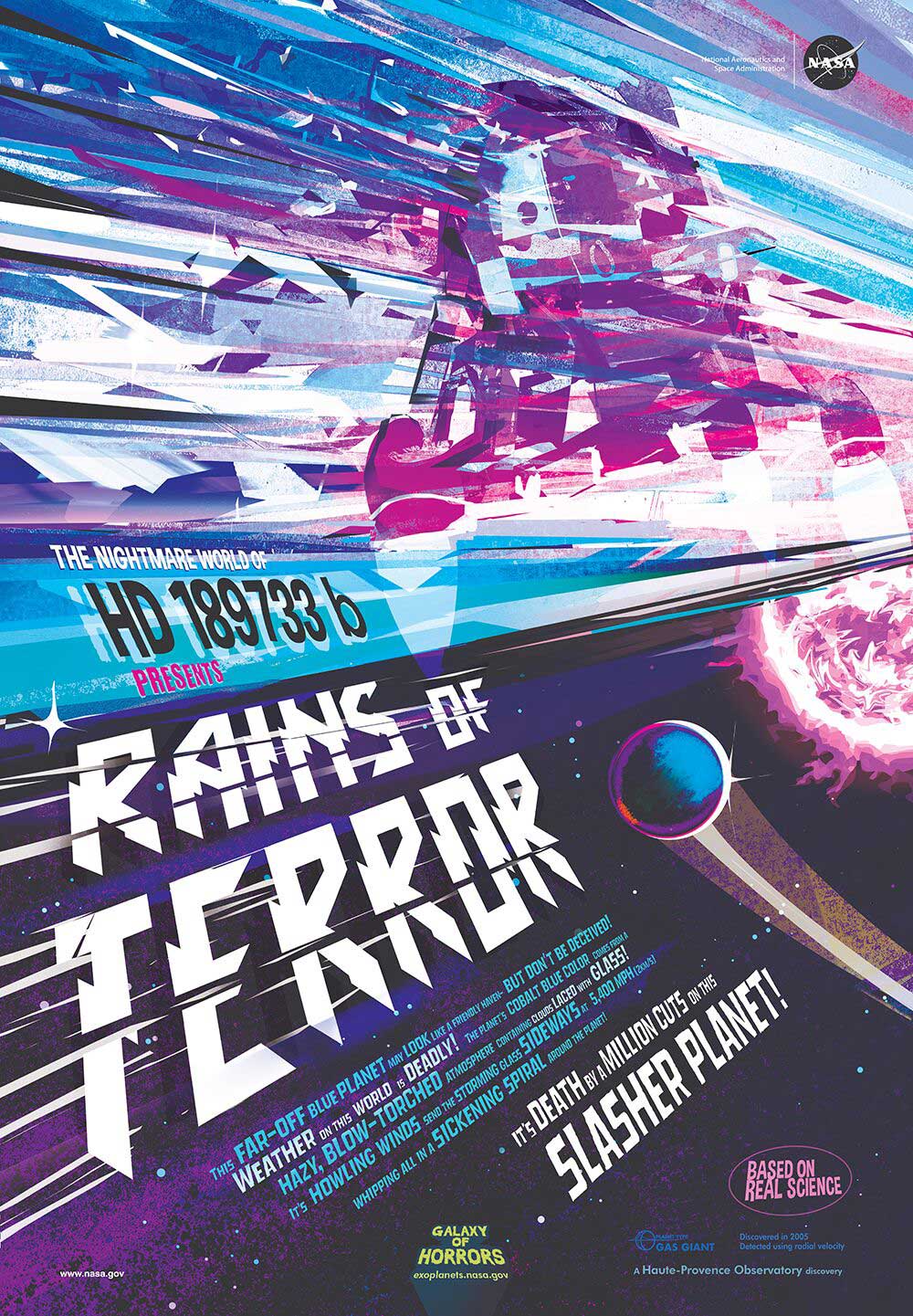This vibrant and striking promotional poster, predominantly in purples, blues, and whites, showcases the terrifying realities of the exoplanet HD 189733B. The vertical rectangular image, devoid of a border or distinctive background, prominently displays a black circle with 'NASA' in white lettering in the upper right corner. The focus is on a depiction of cosmic peril, featuring geometric shapes and a fiery, cosmic ball suggesting a planet or star engulfed in flames. 

Spanning the center left of the poster, the bold white text reads: "The Nightmare World of HD 189733B presents Rains of Terror." Descriptive text details this far-off blue planet, deceptively friendly in appearance, but marked by lethal weather phenomena. The atmosphere, a hazy blowtorch, contains clouds filled with glass, and the howling winds propel the glass sideways at 5400 miles per hour in a sickening spiral, creating a deadly environment where survival is impossible—a true 'death by a million cuts' on this slasher planet. The bottom of the poster, in striking yellow text, features the chilling title "Galaxy of Horrors," alluding to the broader cosmos of fear encapsulated in this otherworldly scene.